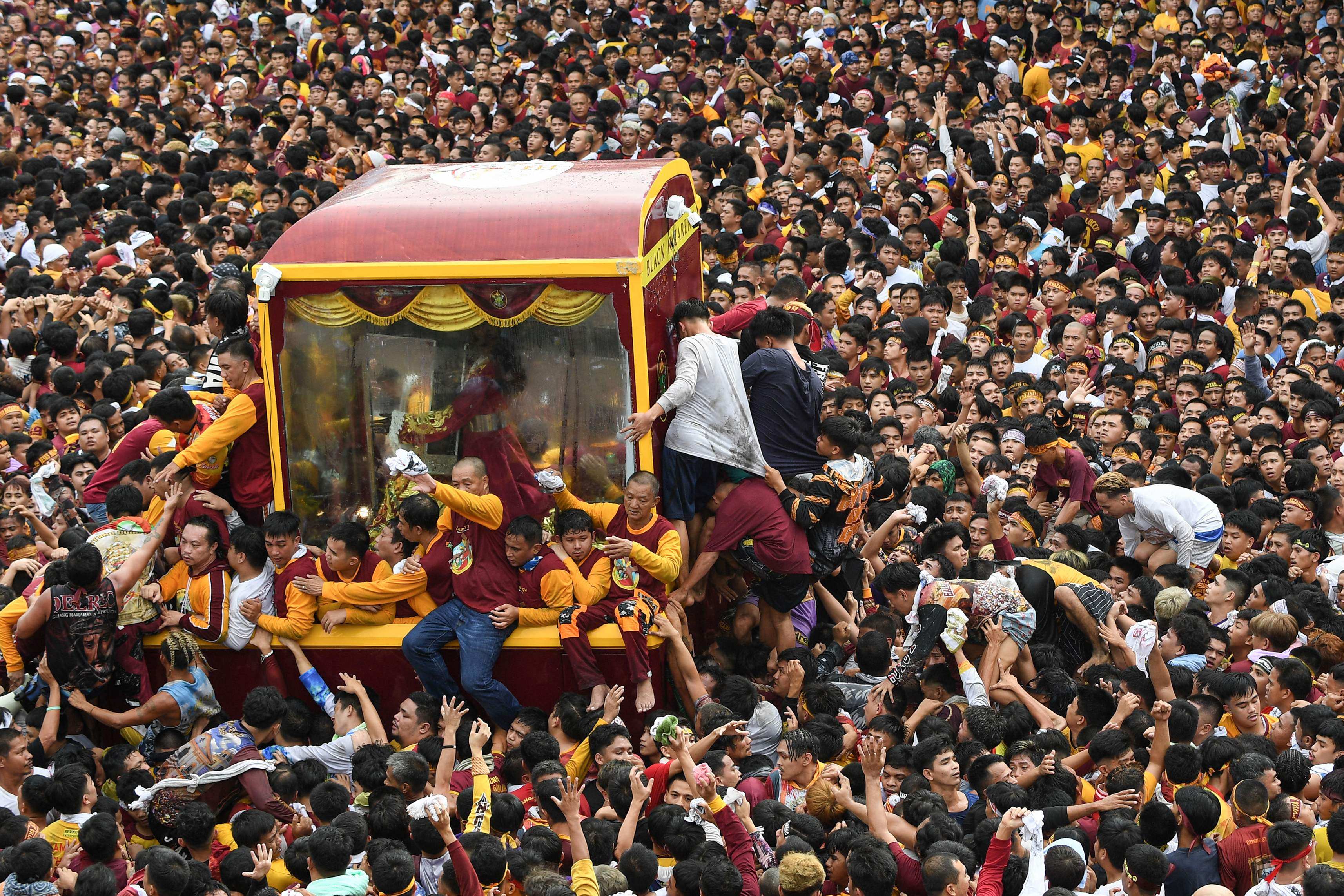This photograph captures a chaotic and vibrant scene with thousands of people packed shoulder-to-shoulder, striving to catch a glimpse of a figure inside a striking vehicle. The vehicle, which is deep red with yellow trim and features a clear glass enclosure, sits slightly left of center in the image. The glass enclosure appears to hold a figure, possibly a famous person or deity, who is standing and waving amidst red curtains. Although the person inside is captured in profile and appears blurry, they are clearly the focal point. Surrounding the vehicle, the sea of people, including what seem to be uniformed men and others attempting to climb onto the structure, create a sense of urgency and excitement. This rowdy crowd, stretching across the image, underscores the significance of the figure inside the glass enclosure and the intense interest they provoke.